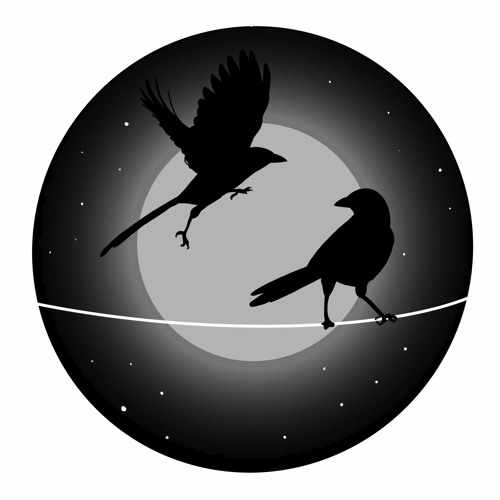The image is a circular vector illustration dominated by black, gray, and white tones. It depicts two silhouetted crows against a backdrop resembling an eye, with a dark outer edge transitioning to a lighter gray center where a light gray moon glows. The sky, forming the 'iris' of the eye, is peppered with white stars. A singular white telephone wire arcs across the lower half of the scene. One crow is perched on the wire, staring at another crow in flight, which appears to be either approaching or departing. This art piece merges the celestial with the terrestrial, encapsulating a moment of avian interaction under a starry, moonlit sky.